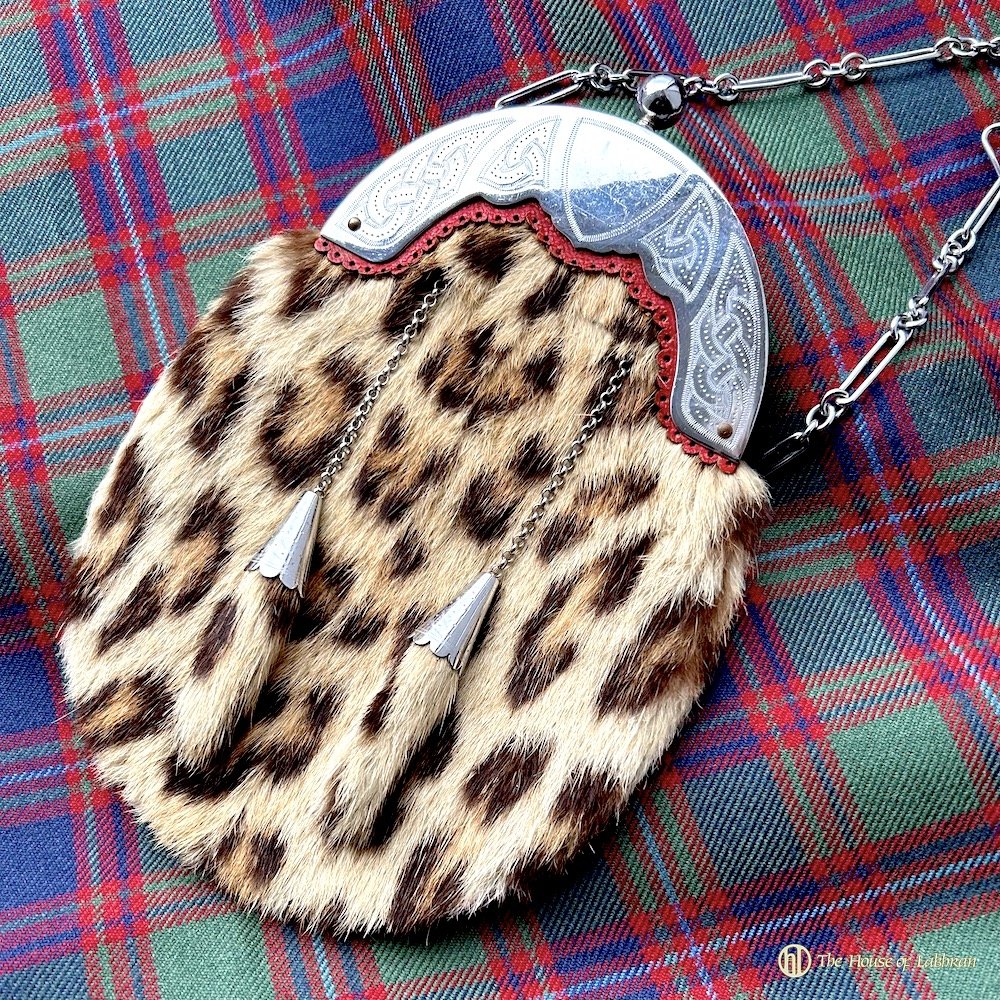This photograph, which is square in shape measuring about six inches by six inches, provides an up-close view of a detailed pouch that hangs from a silver chain. The background showcases a tartan plaid pattern in vibrant red, blue, and green hues, suggesting it might be a kilt. In the lower right-hand corner, there is a gold print emblem featuring a circle with the intertwined letters "H" and "L," accompanied by the text "The House of Labhran."

The focal point is an oblong pouch adorned with leopard-print fur, characterized by distinctive black spots on a blonde fur base, invoking the appearance of a cheetah. The top of the pouch is embellished with a metal plating in a silver or gray steel color, from which the chain extends. Adding to its decorative charm, two additional chains hang down the center of the pouch, each terminating with clumps of matching leopard-print fur, reminiscent of a key charm or a lucky rabbit's foot. The meticulous details of the fur and metalwork, paired with the vibrant plaid backdrop, create a rich, textured scene.